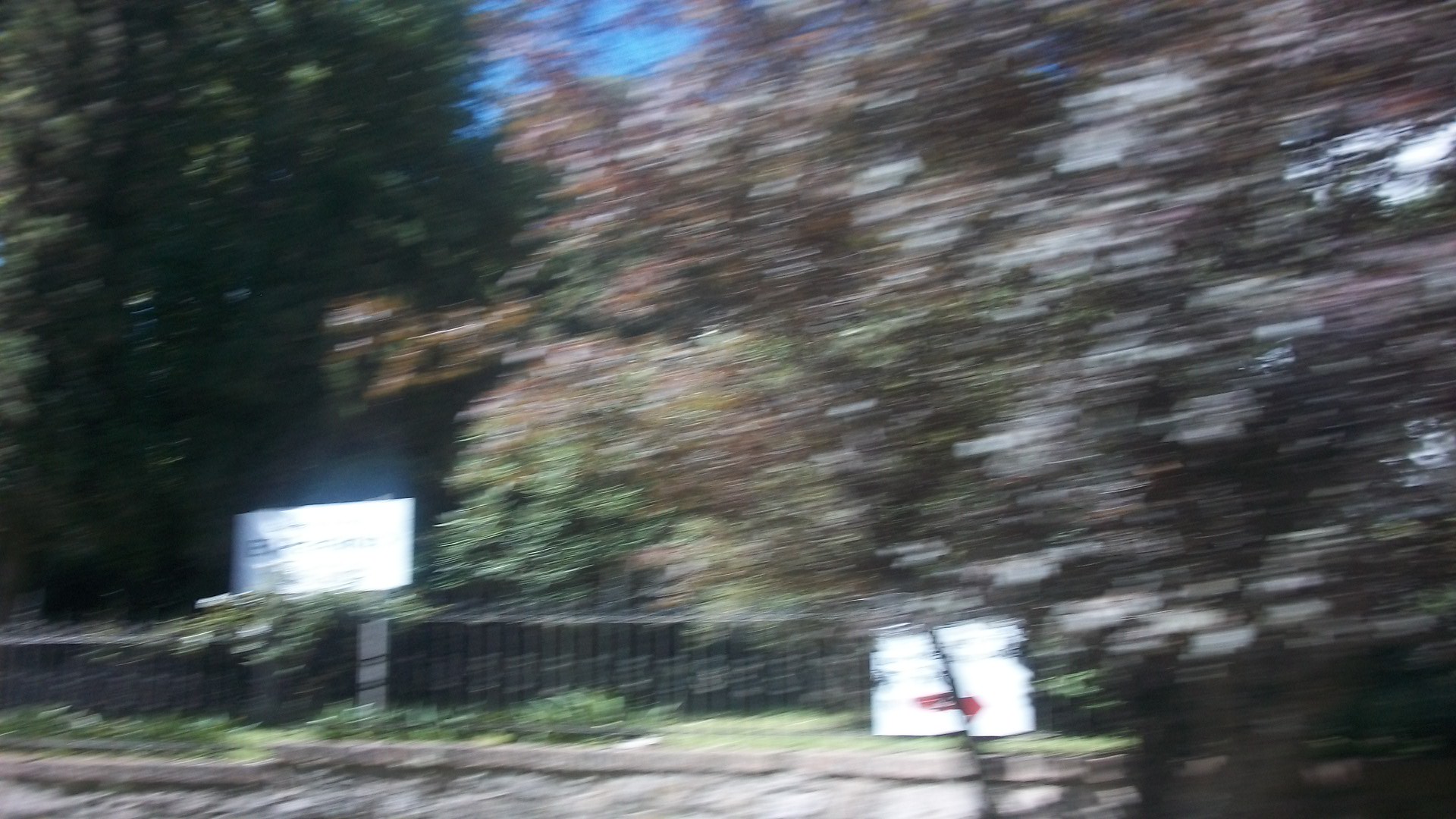This is a blurry photo taken from a camera while in motion, capturing an outside scene rich with trees. Two large trees dominate the foreground: the one on the right has leaves that are a reddish-orange color, while the one on the left has lush green foliage. The background features a mix of near and far distant trees with very bushy branches. Between the trees, glimpses of a deep blue sky indicate it is daytime, possibly approaching sunset. At the base of the trees, there is a short black metal fence encircling what appears to be an establishment. A dark concrete sidewalk runs parallel to the fence. In front of the fenced area, a white board sign is visible on the sidewalk, and to the left, behind the fence, another rectangular yard sign can be seen.